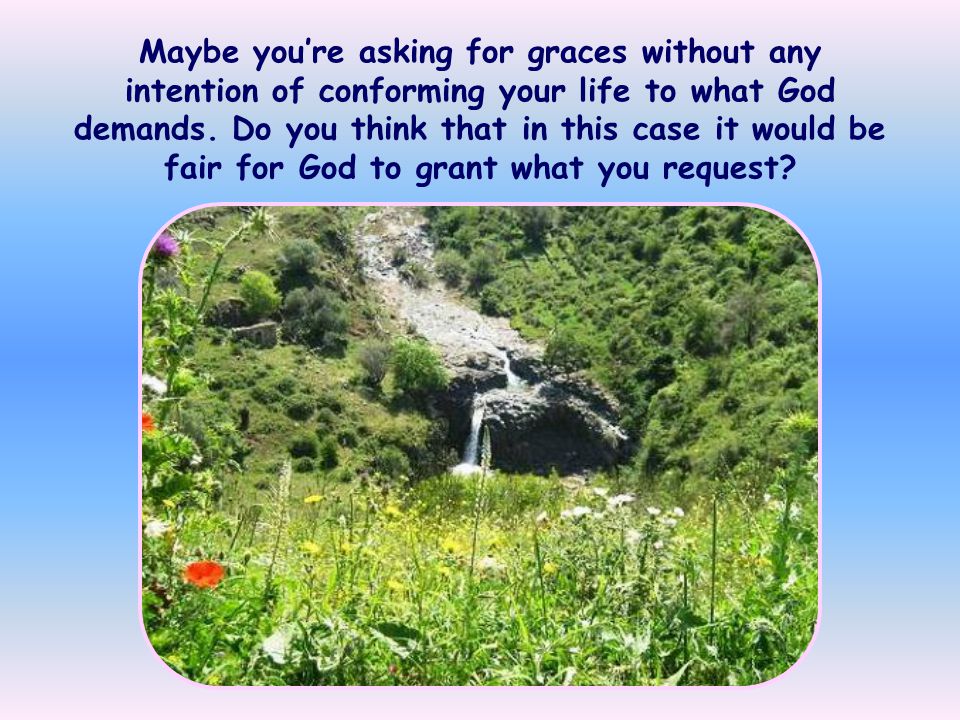This poster, resembling a PowerPoint slide, prominently features a photograph of a serene, natural scene in the center. The image depicts a lush field filled with various types of greenery and an array of flowers, including poppies, possibly daturas, and spiky flowers. A distinctive cave-like structure emerges from the middle of the field, stretching upwards along a hill that ascends towards the top of the photograph. A waterfall can also be faintly seen in the background, adding to the tranquil ambiance of the scene. Surrounding the photograph is a border with a gradient background transitioning from blue to pink. Positioned above the photograph is a reflective message in black text: "Maybe you're asking for graces without any intention of conforming your life to what God demands. Do you think that in this case it would be fair for God to grant what you request?" The poster combines calming visuals with contemplative text, designed to evoke introspection about one's spiritual requests and the harmony of nature.